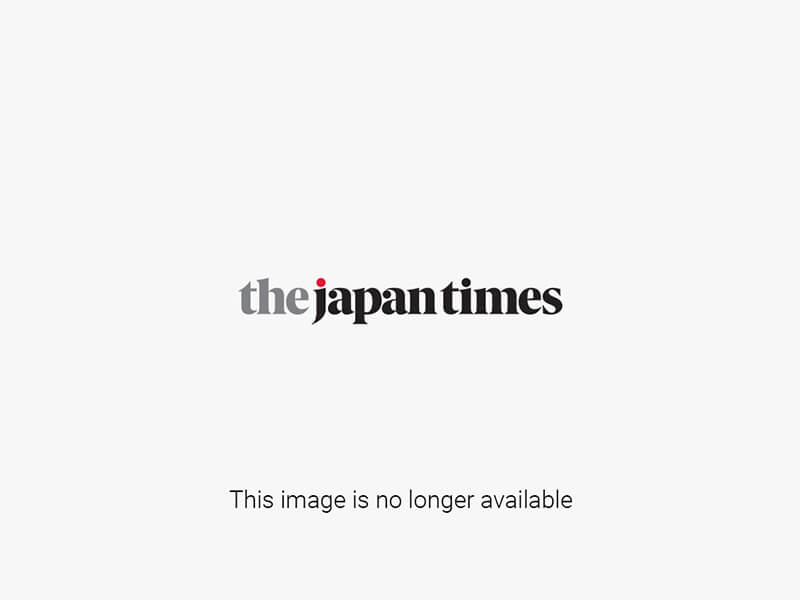This photograph captures a bustling moment at a subway station in Japan. Centered in the image, a two-car train rests at the platform. In the immediate foreground, three women draw attention; two of them have their hands extended, engaged in an animated interaction as they stand close to the wide yellow safety line marking the platform's edge. The scene is framed by large, round white cylindrical supports and a ceiling adorned with a mix of black recessed lighting and fluorescent fixtures, casting a steady glow over the area. Intriguingly, the train cars exhibit two young women climbing out of the windows of the car closest to the viewer, on the left-hand side. In the background, a crowd of commuters fills the scene, with several women walking on the right-hand side behind the support columns, adding to the sense of dynamic movement that characterizes the station.